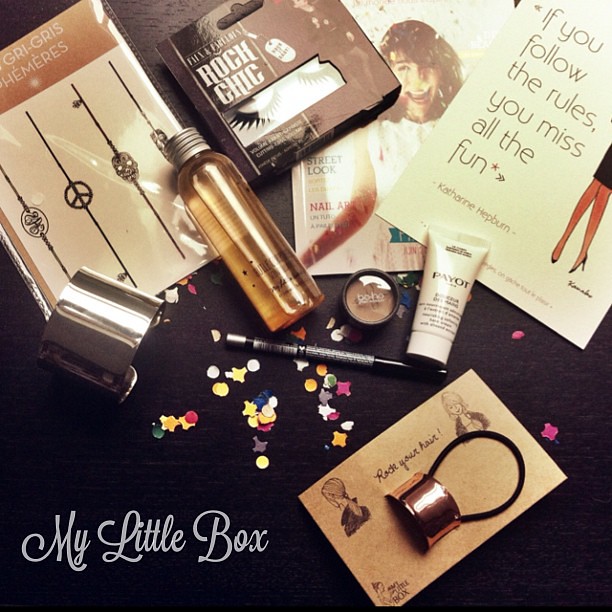The image is a beautifully curated album cover art set against a sleek black background, titled "My Little Box" in elegant script at the bottom. The arrangement prominently features various vintage-inspired beauty and fashion items reminiscent of the 1960s and 70s, all adorned with colorful confetti strewn about the surface.

On the top left corner, a package contains four distinctive bracelets, each adorned with symbols like a peace sign and a sugar skull, evoking the counterculture spirit of the era. Adjacent to it in the center top is a box labeled "Rock Chic," containing false eyelashes, while directly below it lies a magazine with visible headlines "Street Look" and "Nail Art," indicating its focus on fashion and beauty trends.

Overlapping the magazine slightly is an inspirational card with a quote attributed to Katharine Hepburn: "If you follow the rules, you miss all the fun." In the middle of the image, a collection of beauty products stands out: a bottle of clear liquid, possibly perfume or bubble bath, next to a light brown pot of makeup branded "Boho." Beside these is a white squeeze bottle labeled with the logo "PAYOT," commonly associated with skincare, flanked by a black and silver eyeliner pencil.

Towards the bottom right, a specialized ponytail holder designed to incorporate a metal cuff for a more stylish hairdo rests in brown packaging branded "Rock Your Hair." The entire ensemble beautifully merges the nostalgia of vintage fashion with modern beauty essentials, encapsulated within the chic aesthetic of an album cover.